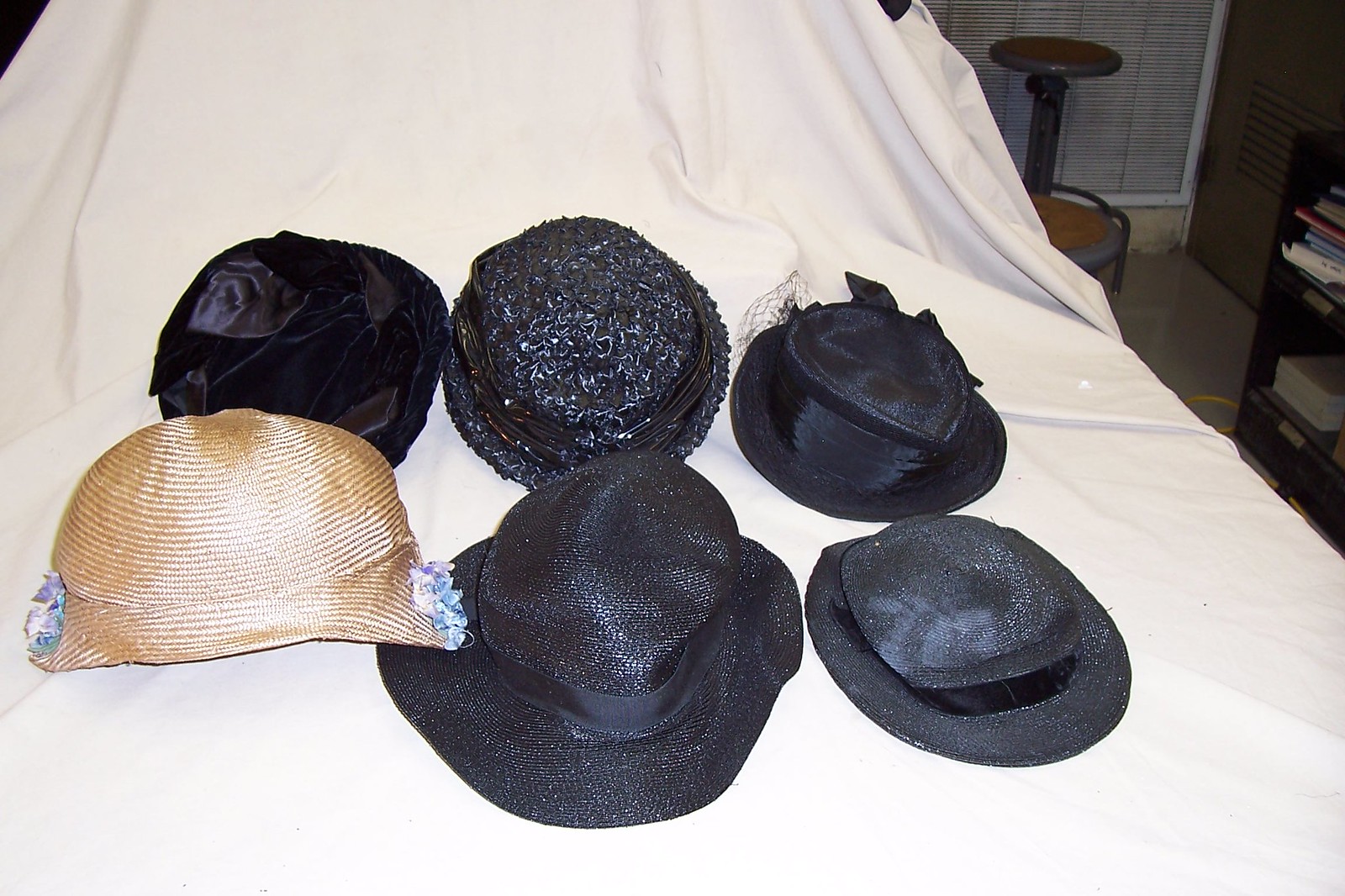In the center of this indoor digital photo, a white linen bed sheet is draped over a bed, providing a backdrop for six elegant vintage hats arranged in a neat three-by-two configuration. Three hats are positioned along the top row and three along the bottom row. In the top row, starting from the left, a black velvet hat with a bow sits next to a textured silver hat with a funky appearance. To the far right, a fancy women’s hat with a satin sheen and a black bow is found. The bottom row features, on the left, a beige straw hat with a short brim. In the center is a wide-brimmed, oversized brown hat with a shiny finish. The bottom right hat is a stylish black hat that appears slightly elevated in style, possibly a crusher type, with a decorative brim.

In the background, a dark black bookshelf filled with various colored books is seen near the upper right corner, adjacent to what seems to be either a gray mini-blind or a textured gray wall. There’s also a small wooden table in brown in front of this backdrop, enhancing the indoor setting of the photo. Furthermore, the upper right corner includes a brown door and a tiny black triangular detail. Clothing the image are various elements of the room, but the main highlight remains the elegant array of diverse vintage hats displayed on the central white bed sheet.